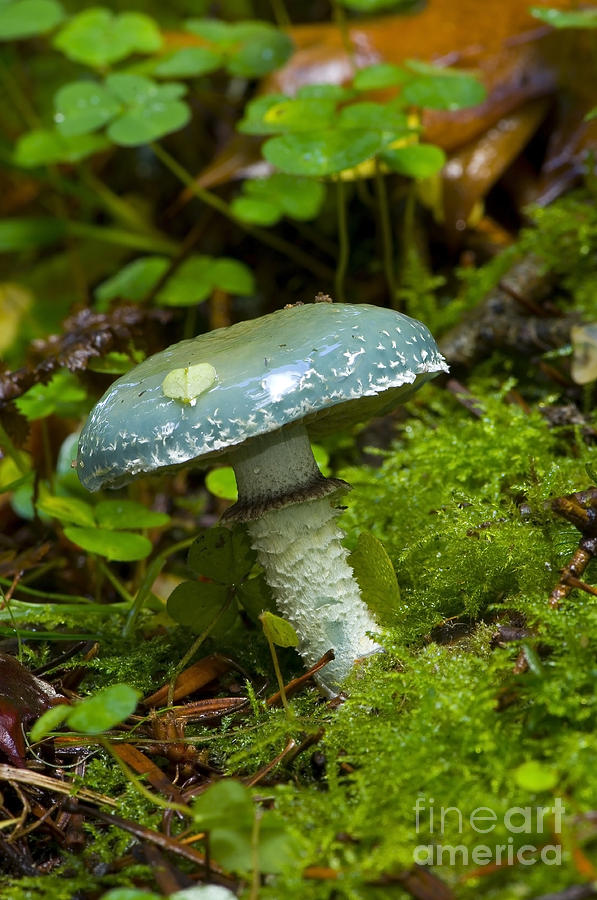In the center of this forest floor scene, a striking blue and white mushroom stands prominently on wet, green terrain. The mushroom's cap is a light blue with white spots and is supported by a thick, mint-green stem. Surrounding the mushroom, the ground is populated with small, green plants, various brown twigs, and scattered dead leaves, creating a moist environment perfect for fungi. Above the mushroom, taller three-leaf clovers, slightly blurry, add depth to the image. In the background, red flowers peek through, adding a touch of vibrant color. Flanking the scene on both sides are dark, wet branches, likely fallen from a nearby tree. Additionally, in the bottom-right corner, a white watermark reads "Fine Art America," subtly identifying the image’s source. The entire scene glistens as though it has recently rained or is covered in morning dew.